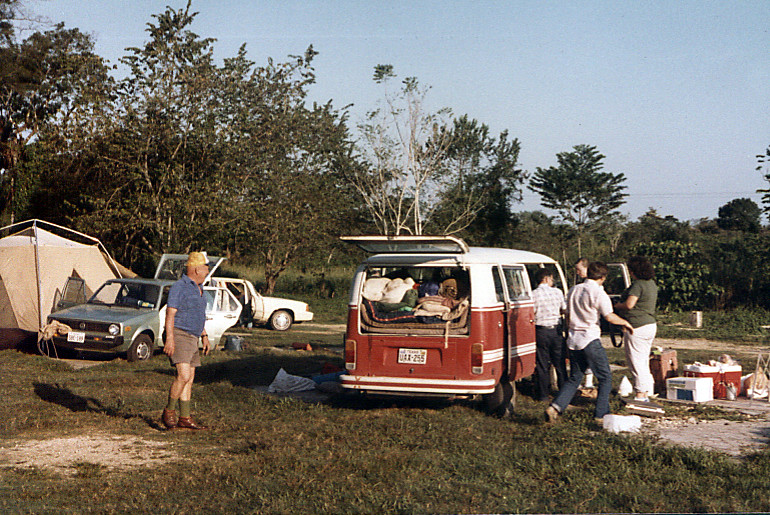This photograph, likely taken in the 1970s or 1980s, showcases a classic red and white Volkswagen microbus at a camping site. The bus, distinct with its red bottom and white top coupled with white stripes on the bumper, has its rear window lift gate and sliding side door open, revealing a collection of camping gear, including rolled-up blankets and pillows. Five individuals are seen around the microbus, busy with packing. To the left, a man in a blue polo shirt, brown shorts, brown shoes, green socks, and a bucket hat is engaged in the process. To the right, another man in a plaid shirt and dark blue pants, a woman in a green shirt and white pants, and two others are organizing coolers and various items near the bus. The grassy campsite is dotted with dirt patches. In the background, two older model cars—a cyan-colored vehicle with its trunk open and a white car with its doors ajar—are parked next to a tan tent with white beams. Beyond the campsite, a tree line stands against a lightly overcast blue sky.